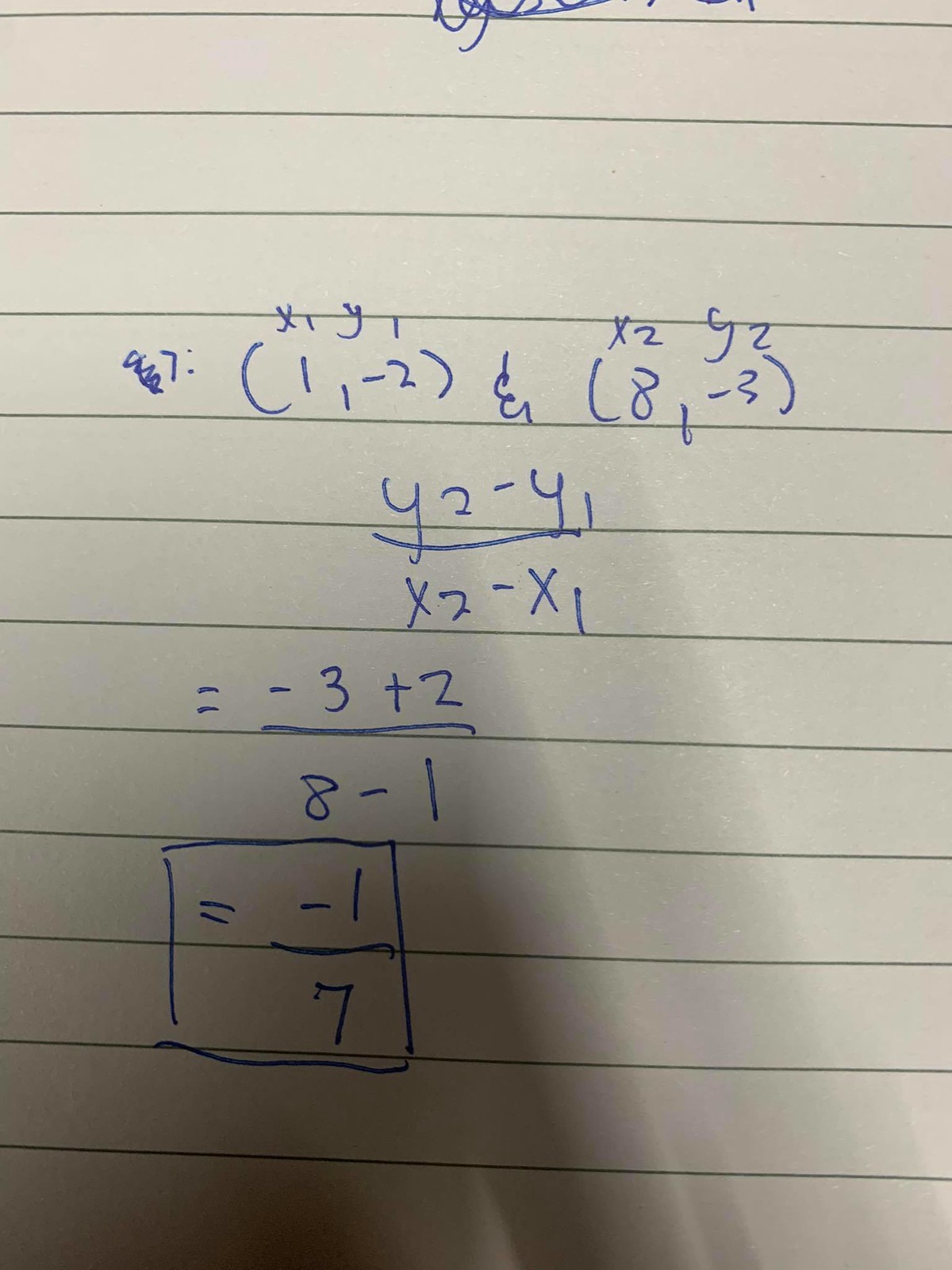This image displays a close-up of a math problem, specifically the seventh equation in a series of calculations. The equation reads as follows: 

\[ \frac{(1 - (-2))}{(x_2 - x_1)} + \frac{(8 - 3)}{y_2 - \frac{42 - 41}{x_2 - x_1}} = 3 + \frac{2}{8 - 1} \]

Enclosed in a box, the equation resolves to:

\[ -\frac{1}{7} \]

In the background, there is the faint outline of a previous equation that has been scratched out and is partially obscured due to the framing of the photo. The rest of the workspace is not clearly visible, keeping the focus on the detailed intricacies of the current mathematical problem.